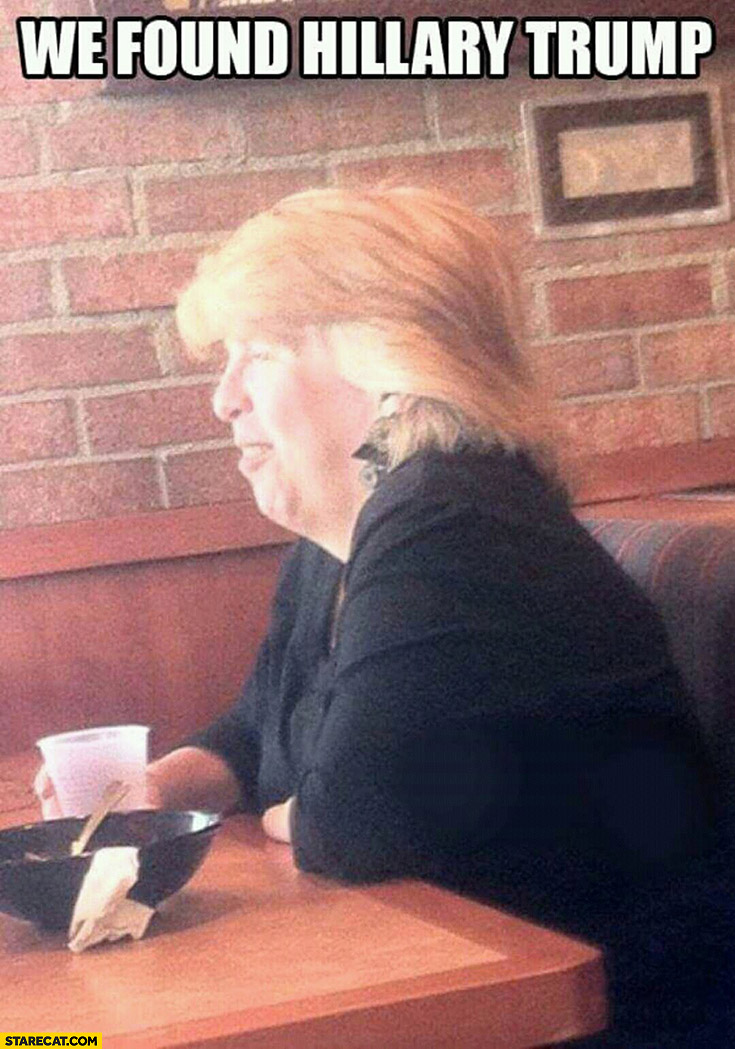The image is a humorous meme captioned "WE FOUND HILLARY TRUMP" in bold, white capital letters outlined in black at the top. The photograph features a woman resembling a blend of Hillary Clinton and Donald Trump. She has light blonde, feathered hair, styled similar to Donald Trump's, and a gullet chin. The woman is seated at a restaurant booth, which has a brick wall behind it and laminated wood features. 

She is wearing a long-sleeved black top, with dangling earrings that combine triangle and circle shapes. The woman appears to be engaged in a conversation, leaning with her elbows on the table and holding a short, translucent plastic cup, which presumably contains beer. In front of her, there is a black bowl with a spoon handle protruding from the right side and a wadded-up napkin partially inside, suggesting she has finished her meal.

The table she's at is two-toned brown, with a dark brown edge and a lighter brown center. A website, "staircat.com," is displayed in black capital letters with a slight yellow border in the lower-left corner of the image. Overall, the meme mockingly combines attributes of both political figures through the woman's appearance and captioning style.